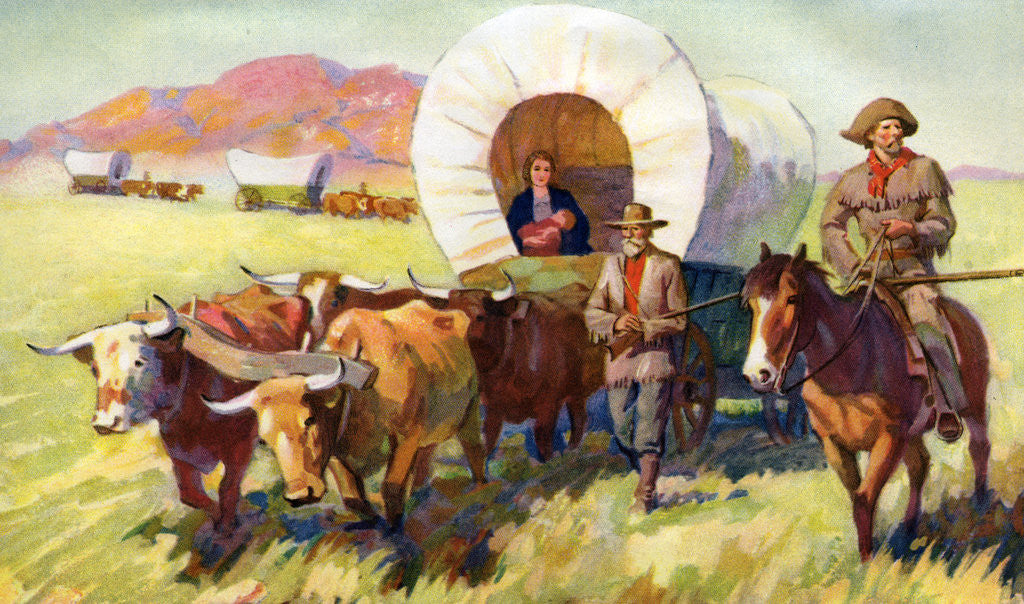The painting depicts a nostalgic scene from the old Wild West, akin to the imagery from the Oregon Trail. Under a hazy daytime sky, the composition features three covered wagons pulled by steers of varying shades of brown, making their way through a vast grassy prairie dotted with gentle hills and towering mountains in the distance.

At the forefront, a woman sits in the lead wagon, cradling a baby in her arms, adding a tender human element to the rugged adventure. Accompanying the caravan are men dressed in hats, some walking beside the cattle, while one elderly man with a gray beard carries a rifle by his side. Another man rides a horse on the right, his rifle resting across his lap as he surveys the scene. The white covers of the wagons billow lightly in the wind, and the entire group seems steadfast in their journey forward, embodying the pioneer spirit of exploration and resilience.